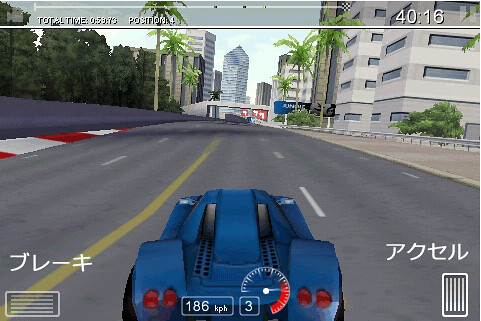A dynamic scene from a video game showcases a sleek, futuristic, slate-blue sports car cruising down an empty road. At the bottom of the screen, white text in a foreign language is displayed on either side. The upper right corner indicates a timestamp of 40:16. The road is marked with a yellow line in the center and white dashed lines demarcating different lanes. Flanking the road on the right are towering corporate high-rise buildings, a wide pedestrian sidewalk, and a protective guardrail. A blue banner, likely from a Marriott hotel, extends from one building toward the sidewalk. The scene is enhanced with numerous palm trees lining both sides of the road, contributing to the futuristic urban setting. Ahead, the cityscape continues with more high-rise structures. On the left, a cement barrier wall stands, with lush tall green trees visible beyond it. The scene captivates with its intricate blend of modern architecture and greenery.